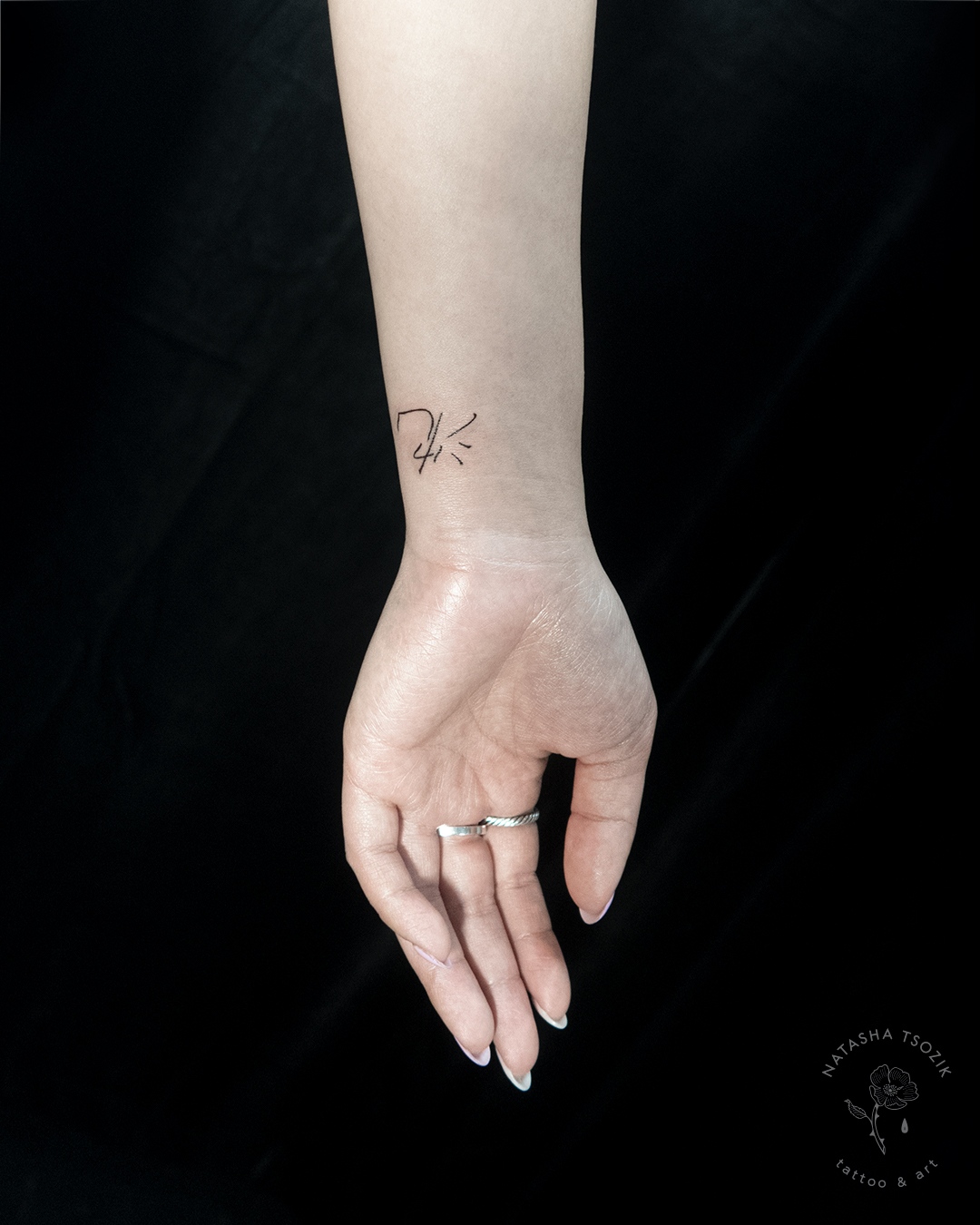The image features a close-up of a woman's right hand, specifically the palm facing up, revealing light skin with a pinkish-gray hue. She is wearing two silver rings on her pointer and middle fingers, and her elongated nails are painted white. On her wrist, there is a small, faint tattoo resembling Asian characters, potentially Japanese, with intricate details such as a '7' base and overlaying '4' with three hash marks extending to the right. The background is black, adding emphasis to the hand and wrist. In the lower right corner, there is a logo that reads "Natasha Tsozic Tattoo and Art," surrounding a rose illustration with a teardrop.